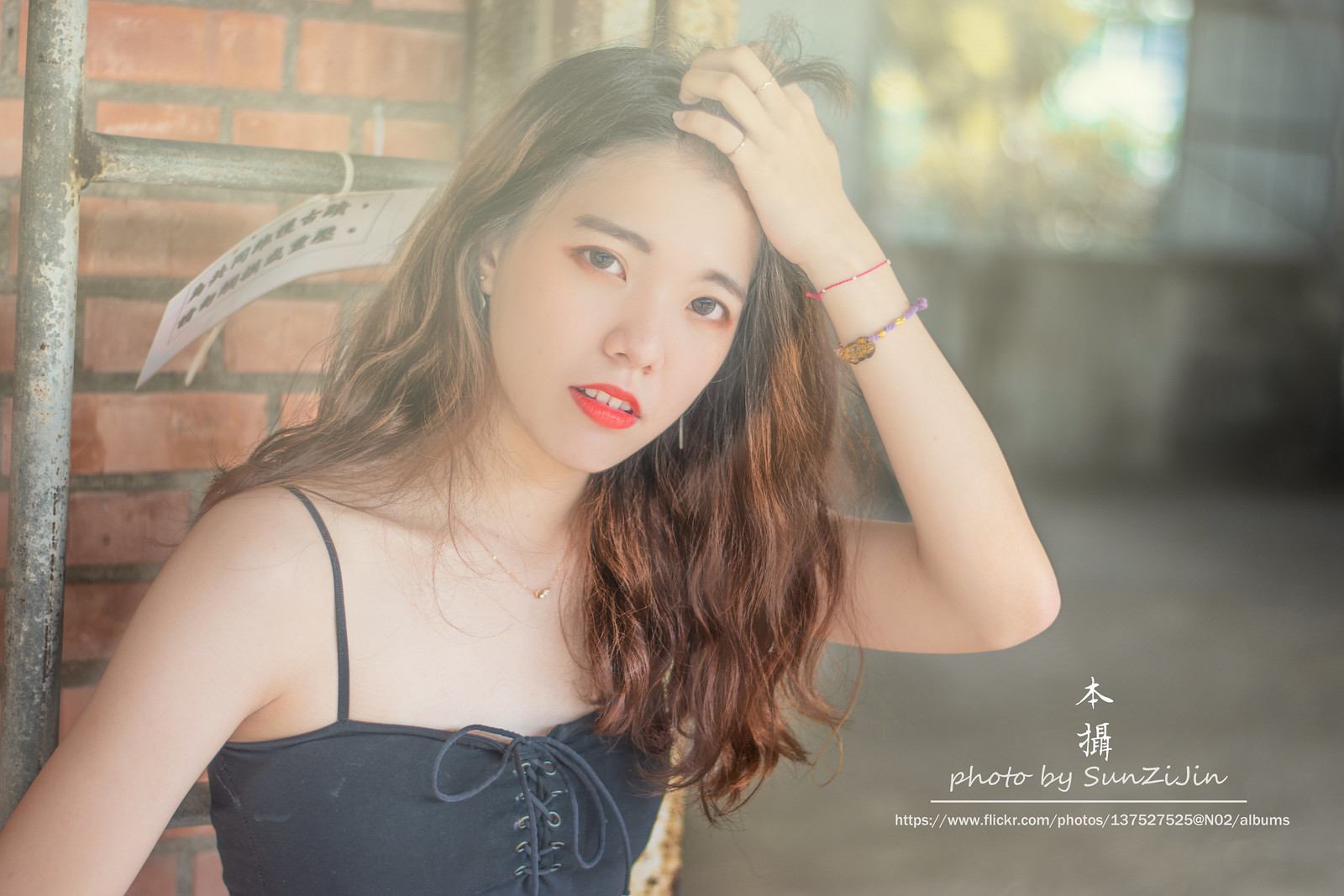The image captures a striking portrait of a young woman standing against a red brick wall. Behind her, a rusty ladder leans against the wall, with a white piece of paper featuring Asian characters zip-tied to it. To the far right, the interior of an industrial building is partially visible, with a concrete floor, metal walls, and an open window that lets light stream into the room.

The woman, positioned prominently in the foreground, gazes directly into the camera, exuding an air of confidence and grace. Her long brown hair cascades over her shoulder, with her left hand delicately running through it. On her left wrist, she wears a pink bracelet and another bracelet with purple and yellow colors. Her left pinky and middle fingers are adorned with identical silver rings. She sports silver dangling earrings and bright red lipstick that adds a pop of color to her look. A gold necklace gleams subtly around her neck.

Clad in a blue dress or top, the photo cuts off just below her chest, leaving the full extent of her attire unclear. In the bottom right corner of the image, there is text in Chinese characters, followed by "Photo by Sun Zi Jin," and an associated Flickr website URL, indicating the photographer's credit and offering a glimpse into their portfolio.

Overall, the portrait is not only a testament to the woman's beauty and style but also subtly serves as an advertisement for the photographer, Sun Zi Jin. The combination of industrial elements in the background with the woman's poised demeanor creates a compelling and detailed visual narrative.